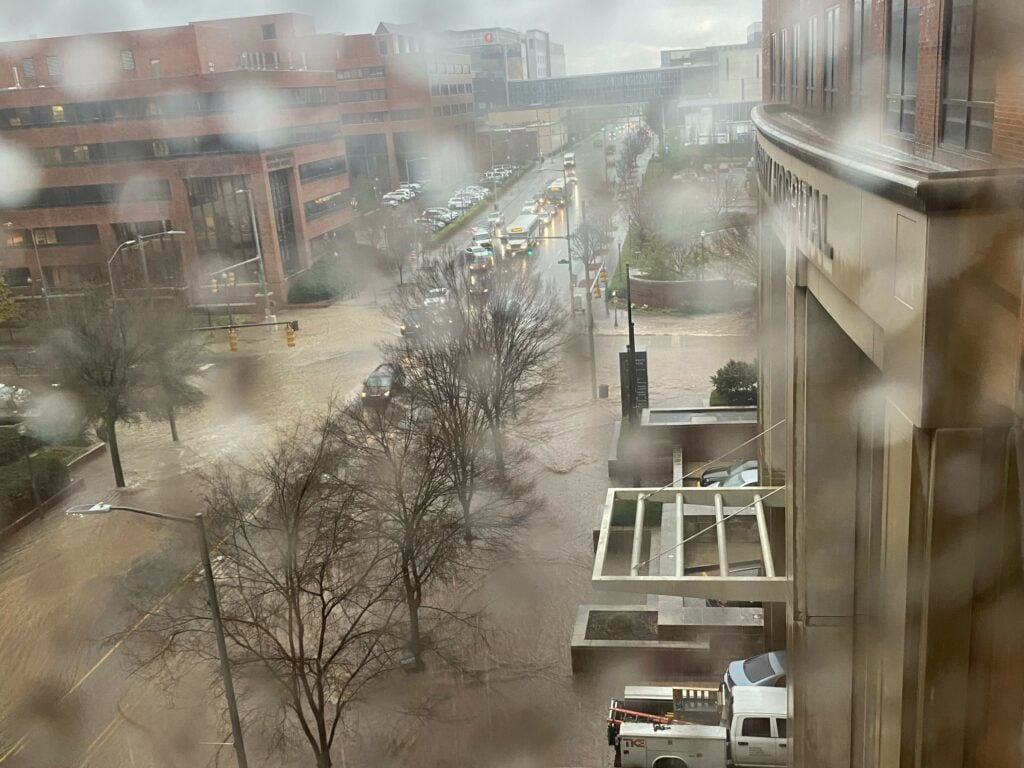This color photograph captures a flooded downtown street from the perspective of a window several stories up in a building, possibly a hospital. The window is spattered with out-of-focus water droplets, indicating it's rainy and overcast. The lens captures a broad view of the cityscape, detailing multi-story, reddish-brown buildings and interconnected glass walkways.

The street below is heavily flooded with brown water, forming several feet deep and engorging the sidewalks and parts of the roadway. The floodwaters have surpassed the median and are only held back in a small, thin area. Cars and trucks are backed up, struggling to navigate the submerged road. On the right side, the large building facing away from the camera displays the word 'hospital', while a truck is stationed at the bottom right corner.

To the left, a significant portion of the highway is underwater, and a line of cars is seen attempting to cross the least flooded sections of the road. The central median is lined with trees, and additional trees are dispersed on the sidewalks and further in the background. Overall, the image poignantly captures the impact of the flooding on urban life, without any visible people present.